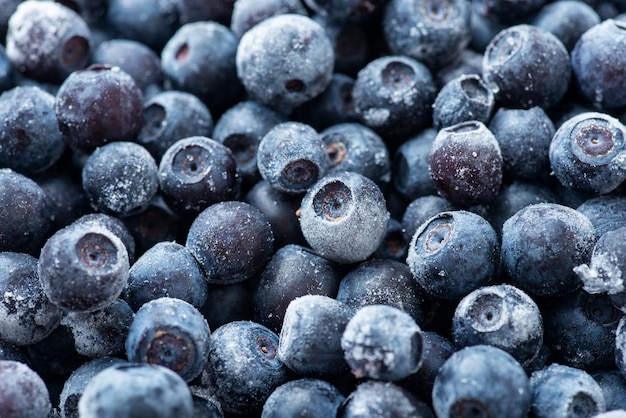The image features an abundant pile of hundreds of blueberries, captured in a top-down view with no visible container or background. Most blueberries exhibit a spherical shape with darker blue centers and characteristic small circular indentations with even darker holes in their centers. Many also have a lighter yellow ring around these holes. The berries, varying slightly in size but predominantly blue to light blue in hue, are coated with a noticeable layer of white frost or possibly fine powder, adding a frosty appearance. A standout among them, situated in the middle of the pile, is a larger blueberry heavily frosted at the bottom. In the upper left, there's another notable blueberry covered in thick white frost with a large, oval-shaped black hole. Some berries are facing upwards, while numerous others are turned upside down, enhancing the texture and depth of the overall composition.